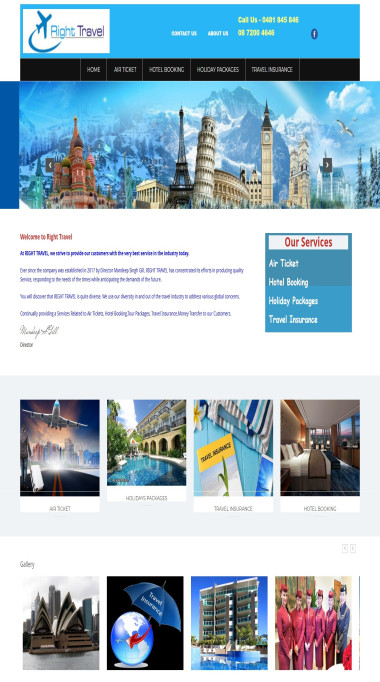The screenshot displays the homepage of the 'Right Travel' website. Dominating the upper right-hand corner is a blue banner featuring a darker blue circle with an exclamation point inside it. Adjacent to this banner, "Call us" is prominently displayed in yellow font alongside a yellow phone number. 

On the upper left side of the image stands the 'Right Travel' logo, set against a white background, which incorporates an illustration of an airplane. Beneath the logo, a black header bar stretches across the top of the page, featuring navigational buttons labeled 'Home,' 'Architect,' 'Hotel Booking,' 'Holiday Packages,' and 'Travel Balance.'

Immediately below the header is a striking, albeit clearly photoshopped, collage image that melds famous landmarks from around the world into one visual. Included in this image are iconic sites such as Big Ben, the Leaning Tower of Pisa, the Eiffel Tower, and St. Basil's Cathedral.

Further down on the webpage, there is descriptive text accompanied by a side banner titled "Our Services." Below this section are several smaller images depicting various travel destinations you can explore through the website.

Overall, the layout is designed to entice and inform prospective travelers with a blend of vivid imagery, essential contact information, and easy navigation options.